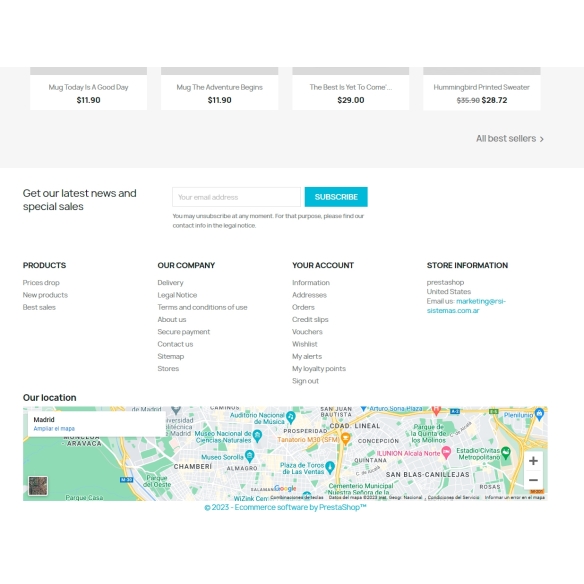The image features a gray top bar containing four distinct sections. Each section houses a white box with a dark gray line at the top. 

1. The first box displays the text: "Today is a good day." Its price is listed as $11.90.
2. The second box states: "Mug - The Adventure Begins," also priced at $11.90.
3. The third box reads: "The Best is Yet to Come," and costs $29.00.
4. The final box showcases: "Hummingbird Printed Sweater," previously priced at $35.90, now marked down to $28.72. Below this box, there is a label that reads "All Best Sellers."

The bottom half of the image consists of a white section. On the left-hand side, there is a prompt that says, "Get our latest news and special sales." To the right, there is a text input box meant for entering an email address, accompanied by a blue "Subscribe" button.

Further down, there are four vertical columns labeled as follows:
1. Products
2. Our Company
3. Your Account
4. Store Information